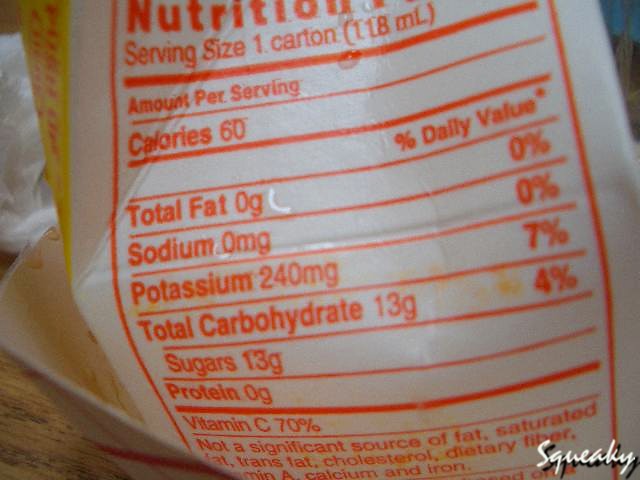This image depicts a realistic close-up photograph of a food product with its nutritional information prominently displayed. The focus is on the back of a white packaging, possibly a juice carton, with orange text detailing the nutrition facts. The background consists of a light tan hardwood surface on the bottom left, adding a warm, natural contrast. Situated within a white bowl or similar container, the packaging reveals key nutritional information: serving size is one carton (118 ml), with 60 calories, 0 grams of total fat, 0 milligrams of sodium, 240 milligrams of potassium (7% DV), 13 grams of total carbohydrates (4% DV), 13 grams of sugars, 0 grams of protein, and 70% of the daily value for vitamin C. The nutritional information is clearly formatted, making it easy to read. In the lower right corner of the packaging, the word "squeaky" is written in white font with a black shadow. The detailed nutritional facts and practical design suggest the product could be a form of juice, although the photo does not show the front or contents of the packaging.